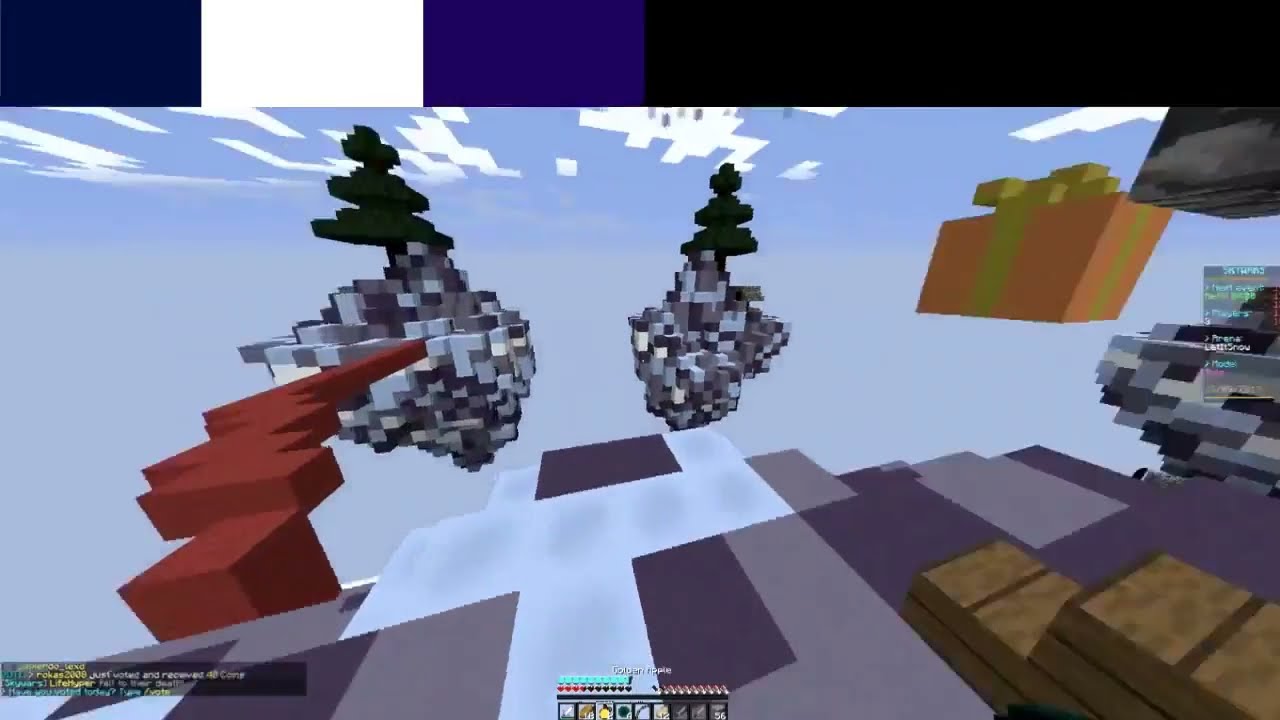The image is a still from a video game, reminiscent of Minecraft, with cartoonish, pixelated graphics. The sky is light blue with digitized white clouds, and a large orange present with a yellow ribbon floats in the upper right corner. The scene features a red pathway on the left, bordered by steps ascending into the distance. This pathway leads to floating blocks with sculpted, spiraled trees growing out of them. 

On the right side of the image, two light brown rectangular platforms are stacked on top of each other, resting on a combination of purple and grey pathways. Above them, a cluster of gray, black, and white objects is piled up, resembling an intricate structure made of cubes and rectangles. 

The foreground contains flat, long brown boards, and there are floating chunks of rock with trees on them, suspended mid-air towards the center of the scene. The bottom part of the screen displays text on the left and middle, alongside indistinct menu options. The top border features a sequence of horizontal rectangles in black, blue, and white.